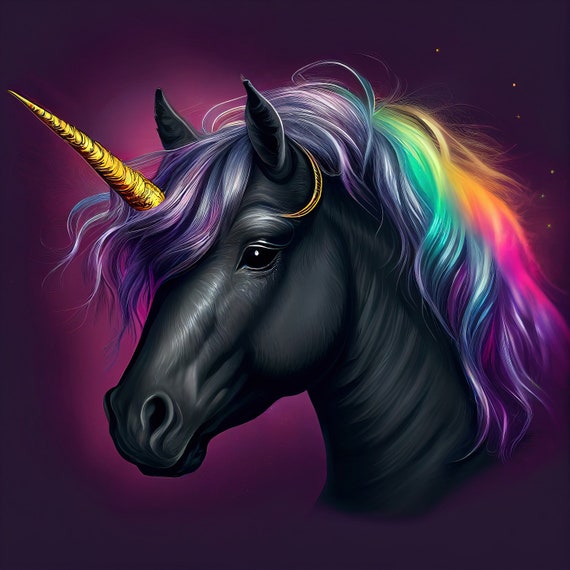The image is an AI-generated or computer-generated square artwork featuring the head and neck of a unicorn. The dark purple and black background gradually lightens to a lighter purple towards the center, where the unicorn is featured. The unicorn, depicted in a side profile with only the left side of its face visible, has a black head and neck, contrasting with the typical white depiction. A golden horn protrudes from between its eyes, angled towards the top left of the image. The unicorn's thick, flowing mane cascades over its face like bangs and trails down the nape of its neck, displaying a gradual transition of colors from purple, light blue, green, yellow, pink, to orange. This vibrant mane and the intricate detailing highlight the uniqueness of the piece, focusing solely on the unicorn's head, excluding any part of its body.